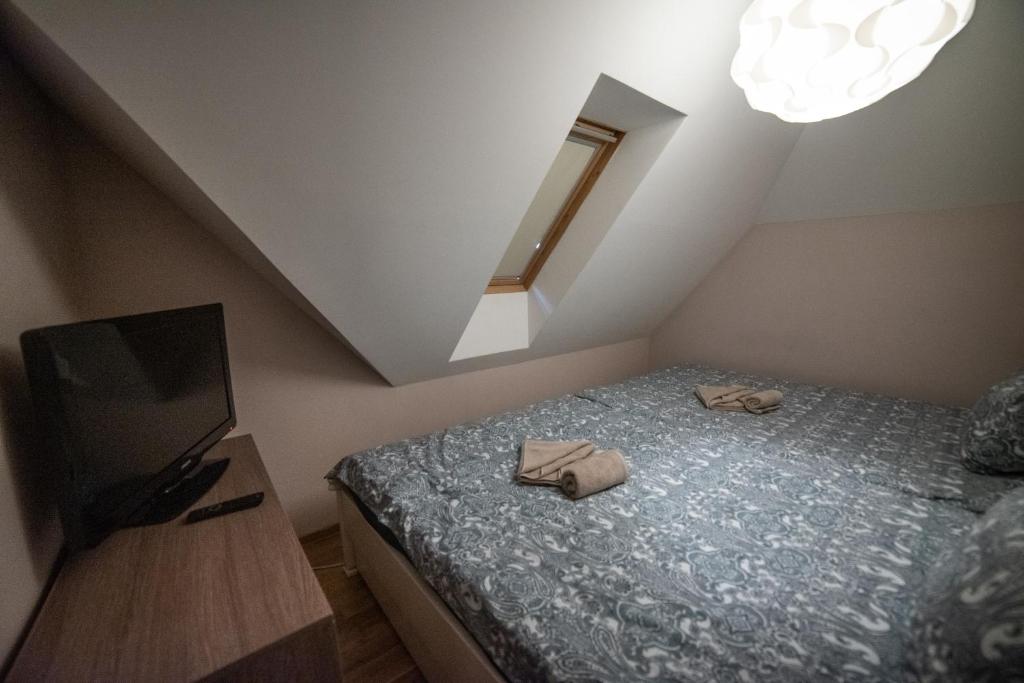This photograph captures an attic-converted bedroom characterized by its cozy, angular architecture. The room's off-white walls emphasize the slanted ceiling that creates a snug atmosphere. Dominating the right-hand side and nearly occupying the entire floor space is a substantial platform bed, adorned with a grayish-blue duvet cover and matching pillowcases. At the foot of the bed, two rolled-up brown towels hint at a bed-and-breakfast vibe. A dark wooden dresser is situated on the left side, supporting a black television with its corresponding remote nearby. Overhead, an intricate scalloped light fixture provides illumination, positioned slightly askew due to the sloped ceiling. Toward the back of the room, an inset small rectangular window punctuates the angled wall, drawing in natural light and adding to the attic's charm.